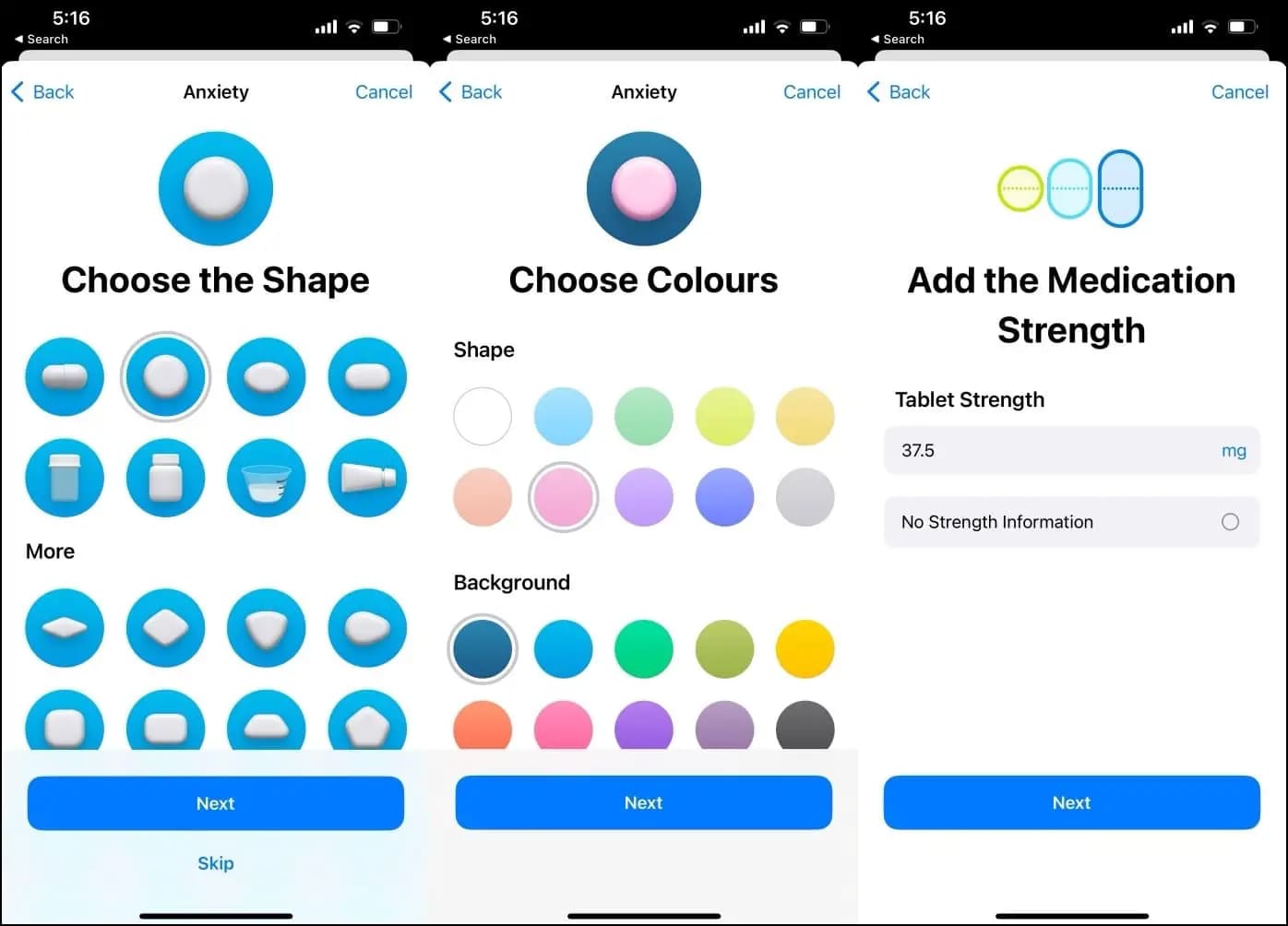The image depicts a detailed medication management system designed to help users customize and keep track of their medications. The interface allows the user to specify various attributes of their medication regimen. Initially, users select the purpose of their medication, with this particular example focusing on anxiety treatment. 

The interface offers a variety of pill shapes including capsules, round, oval, and diamond shapes. It also provides options for different types of containers—clear or solid color bottles, liquid measures, or even cream tubes. Users have the ability to select the color of their pills, with options ranging from white, blue, green, yellow, pink, peach, purple, dark purple, to gray.

Furthermore, users can input the medication’s strength, illustrated here with a chosen dosage of 37.5 milligrams. This comprehensive system aims to facilitate accurate medication identification and adherence, catering to individual user needs.